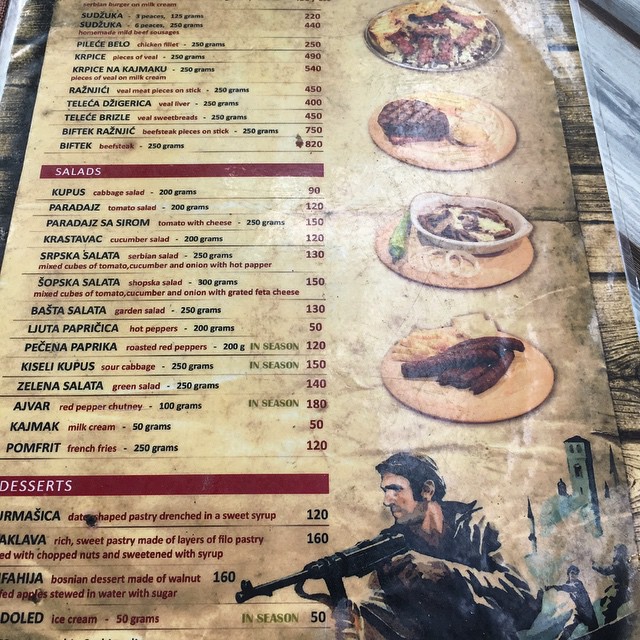This menu photograph features a striking background illustration set in the bottom right corner, depicting a man clad in camouflage green attire, aiming an automatic rifle, with dark hair and a beard. Behind him, medieval buildings and a chaotic skirmish with people fighting on the ground can be seen.

In the central portion of the menu, there are four tantalizing images of various platters and plates of food. Among the clearly highlighted sections are "Salads" and "Desserts." Some notable menu items include "Cupas," "Paradise," "Pasta Salata," "Zalina Salata" (which translates to green salad), and "Pomfret" (french fries). The menu items are listed in both a native language and English, with the English titles clearly displayed beside the translated names.